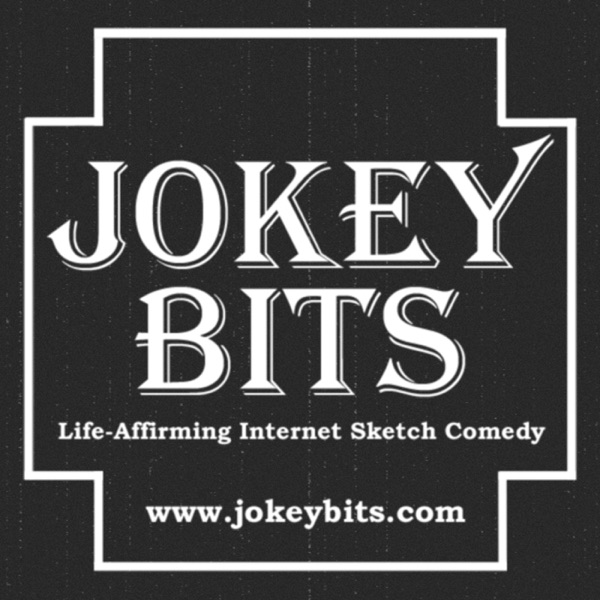The advertisement features a nearly black background with a slightly lighter shade, creating a subtle contrast. Central to the design is a unique white border resembling a fat plus sign or an indented square, emphasizing a centered text. The prominent text within this border is neatly organized in three sections. First, in large, all-capital white letters with a 3D effect, it reads "JOKEY BITS." Below this, in smaller, standard white font, the phrase "LIFE AFFIRMING INTERNET SKETCH COMEDY" is displayed. At the bottom, the website "www.jokeybits.com" is clearly listed in white. The overall presentation suggests a sophisticated, minimalist design for an internet sketch comedy brand.